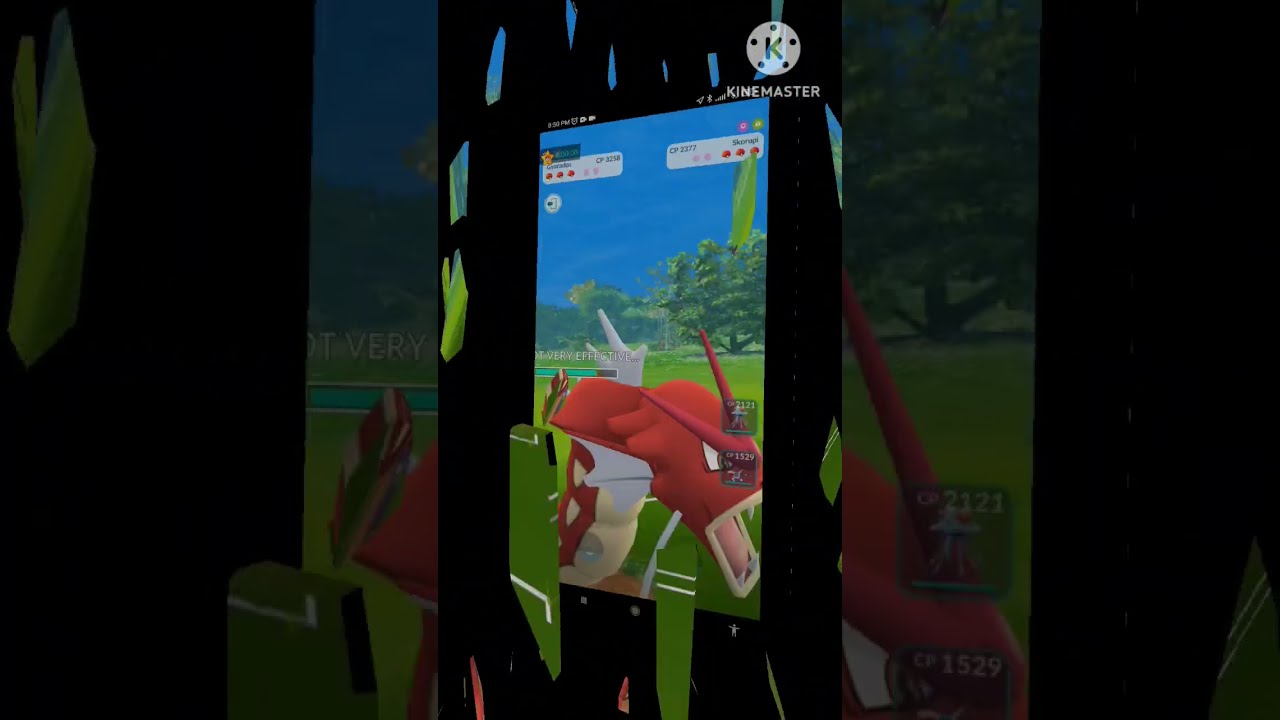The image is an illustration of a smartphone screen displaying an animated scene that appears to be a screenshot from a game featuring a red dragon-like creature with white eyes, pointy horns, sharp fangs, and a pink tongue sticking out of its open mouth. The creature, which may resemble a dragon-type Pokémon like Gyarados, is situated on a green football field with trees and a dark blue sky in the background. The scene has elements that suggest it is part of a competitive video game interface, including icons and what might be a health bar and a count of Pokeballs in the game. The main image is flanked on the left and right by faded, zoomed-in segments of the same central illustration, creating a banner-like effect. Confetti-like shapes in blue and green overlay a black border framing the entire scene. In the upper right corner of the image, the text "KineMaster" is visible, suggesting the use of editing or streaming software.